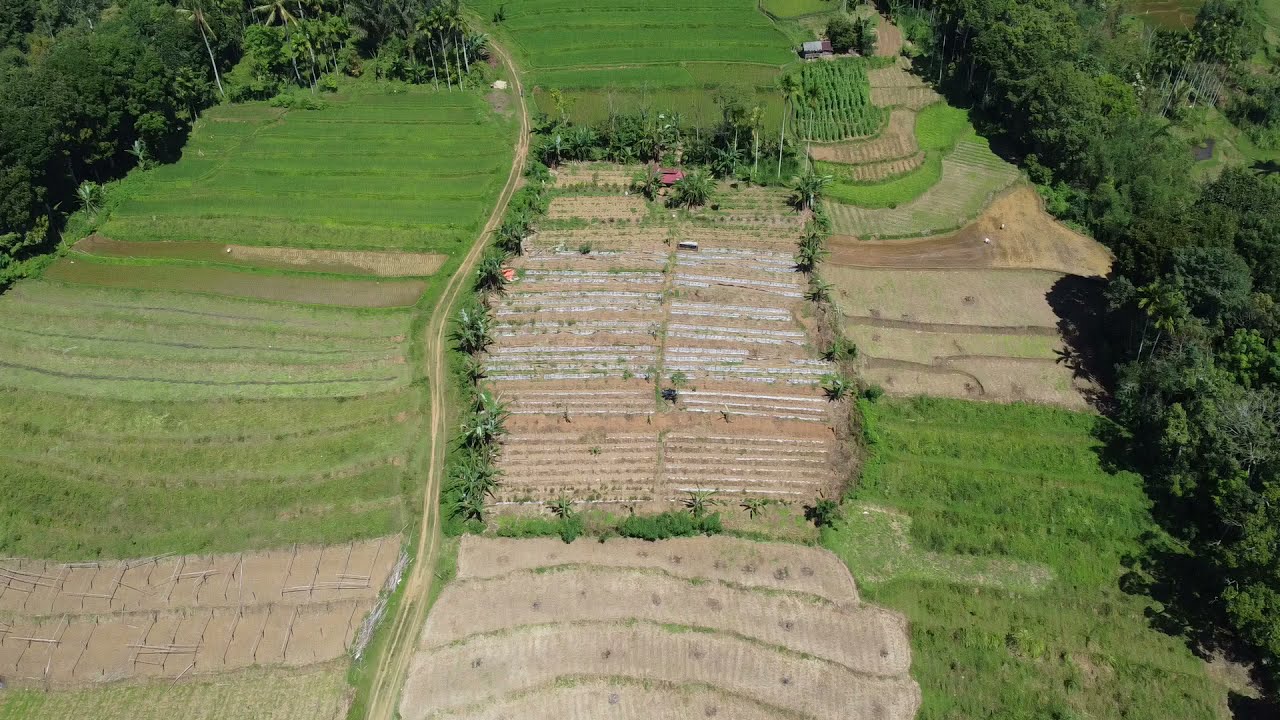This aerial image showcases a lush, green agricultural landscape dominated by a rectangular field at the center. This field is segmented into horizontal rows, likely dedicated to various vegetable crops, and is surrounded by dense, diverse plant life. To the left of this cultivated area, a slightly winding dirt road stretches vertically through the scene. On either side of the road, the terrain is mostly flat with patches of greenery and areas that appear to be unplanted or yet to grow. Flanking the top left and right edges of the image are woods with trees boasting thick foliage in various shades of green, adding to the vibrant scenery. Notably, there are some pieces of farm equipment visible, including a red tractor or building in one of the front fields, and a small structure situated beyond what appears to be a corn field. The overall image captures a thriving agricultural hub with both cultivated and untapped potential.